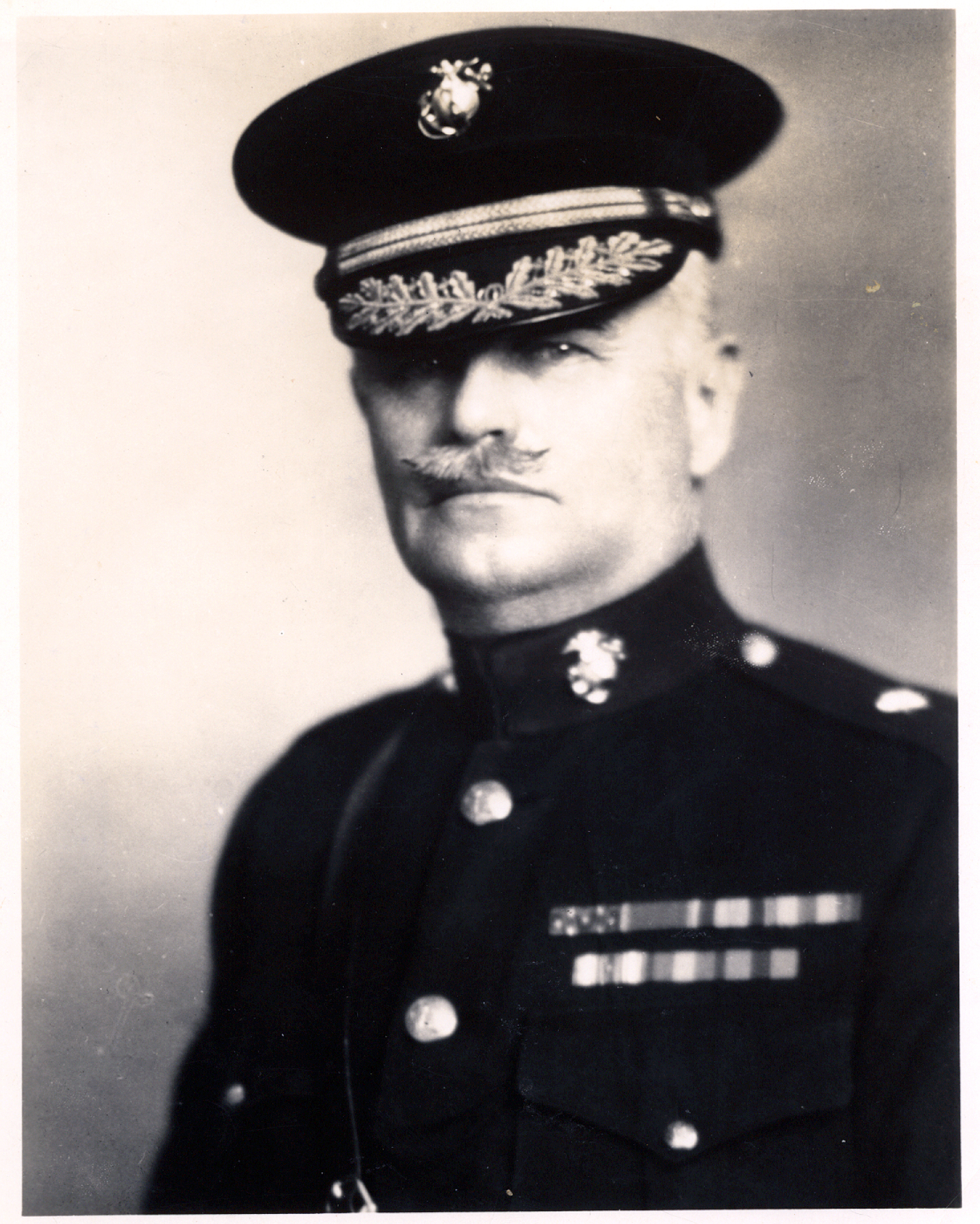This black-and-white portrait photograph features a solemn-looking military general, possibly from the Marines or Navy, outfitted in his formal uniform. He sports a neatly trimmed mustache and well-groomed hair. His uniform includes a dark cap with an emblem in the center—a globe with an anchor, indicative of the Marine Corps—alongside intricate leaf-like patterns embroidered on the bill and a rope around the hatband. The uniform is adorned with brass buttons and medallions on the front, with a pocket on the shirt exhibiting his service ribbons. The general stands against a grey background, exuding a sense of discipline and decorum representative of his high-ranking position, potentially alluding to historical figures like General Pershing from World War I.